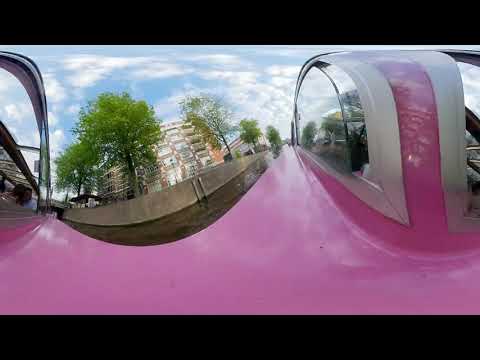The image presents a distorted, fisheye-like view dominated by a pink-hued object, likely a vehicle, possibly a car or bike, with white interior seats and glass windows. The scene appears to be seen from the vehicle's perspective, showcasing multiple elements. In the center of the image, there is a white and reddish-brown apartment building or office building, characterized by balconies and surrounded by tall green trees, five of which are distinctly visible. One of the trees notably has very few leaves. The building is bordered by a dark grey fence with two poles prominently placed at the center. Above, the sky is predominantly blue with scattered white and gray clouds, presenting a mostly overcast atmosphere. The right and left sides of the image are partially obscured by the vehicle's glass windows, further enhancing the distorted, surreal quality of the photograph. A concrete median, appearing brown, is also present in the scene, contributing to the urban environment depicted.